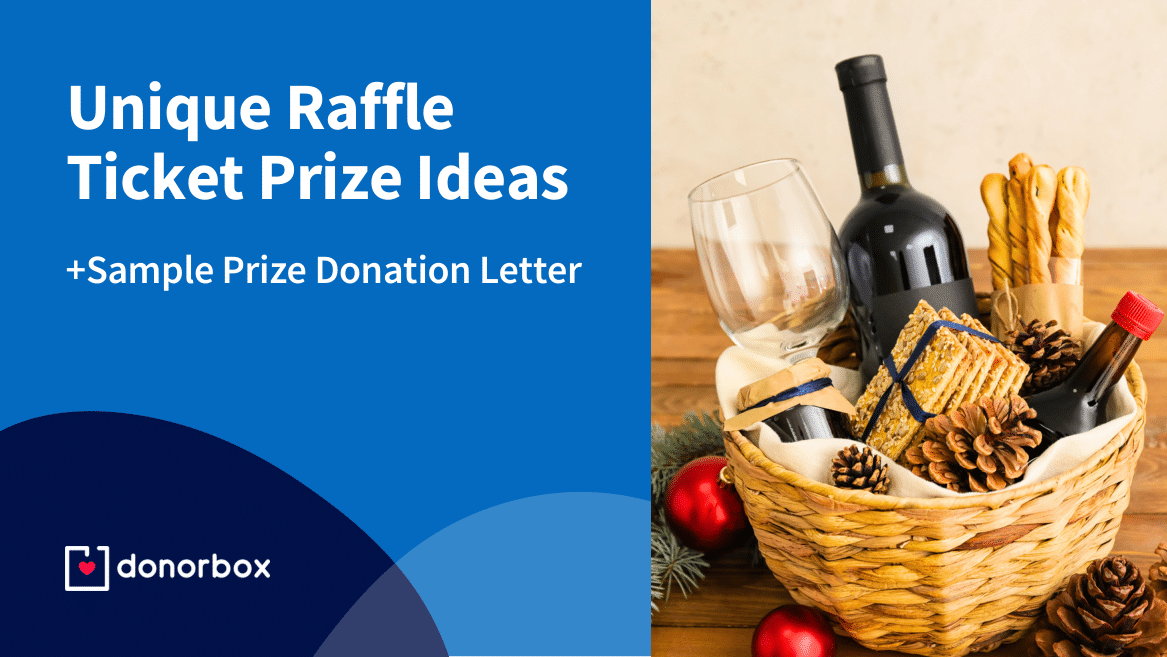This highly detailed promotional image, likely designed for social media or a website, is split into two distinct sections. The left half features a vibrant royal blue square with the caption, "Unique Raffle Ticket Prize Ideas Plus Sample Prize Donation Letter," rendered in crisp white text. Below this sits a navy blue semi-circle containing the phrase "Donor Box" in white letters, accented by a red heart, and accompanied by an adjacent light baby blue semi-circle. The right half of the image showcases a meticulously arranged photograph of a wicker wine basket. This basket is brimming with an assortment of items, including a bottle of wine, a delicately tall wine glass, gourmet seed-topped crackers tied with a ribbon, long breadsticks, and a jar of jam or spread. A light-colored napkin is also nestled inside. Surrounding the basket are festive elements such as red Christmas ornaments, pine cones, and sprigs of greenery, adding a seasonal touch to this appealing raffle prize idea.